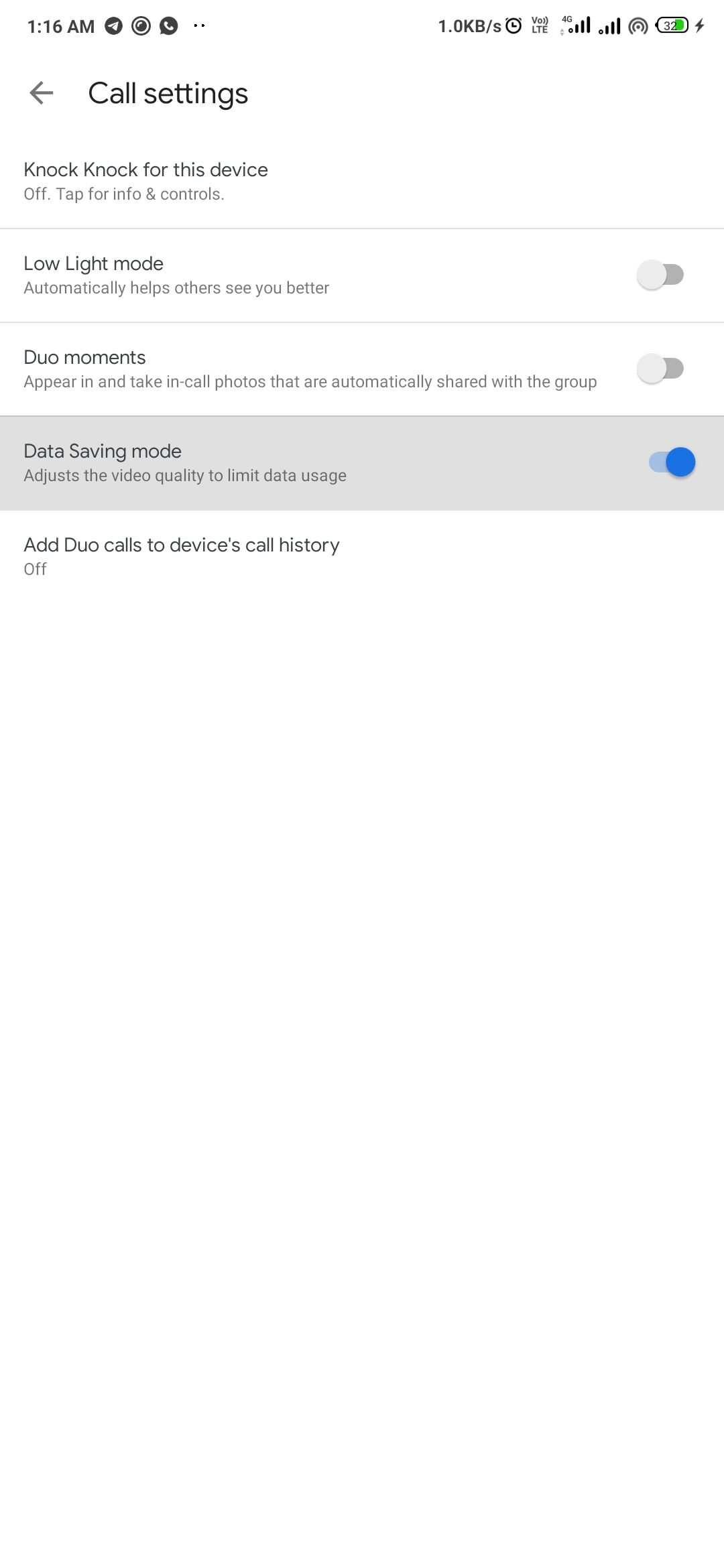Screenshot of a mobile phone displaying the call settings page for the Google Duo app. At the top of the screen, standard phone status icons are visible, including battery usage, time, and wireless network strength. The title of the settings page, "Call Settings," is displayed prominently.

There are five distinct sections listed on this page:
1. **Knock Knock for this device** - This setting is turned off.
2. **Low light mode** - Automatically helps others see you better. This setting is also turned off.
3. **Dual moments** - This option is turned off as well.
4. **Data saving mode** - This setting is activated, indicated by a blue toggle button set to the right and highlighted in dark gray.
5. **Add Duo calls to device's call history** - This final setting is turned off.

The visual difference between active and inactive settings is clearly shown, with the active "Data saving mode" being distinctly highlighted compared to the other settings.